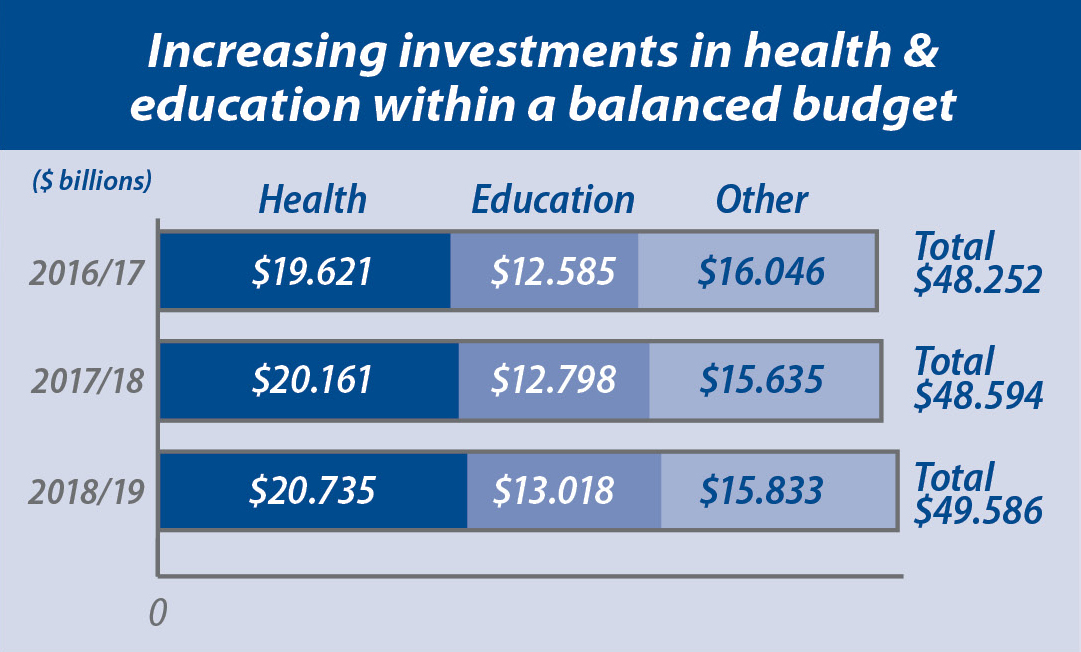The image displays an infographic that resembles a PowerPoint presentation slide, featuring a plain light blue background and a prominent dark blue banner at the top, which states in white text: "Increasing Investments in Health and Education within a Balanced Budget." Below this banner is a bar graph divided by years—2016/17, 2017/18, and 2018/19. Each year's data is presented on the y-axis, with three distinct colored horizontal bars representing spending categories: Health, Education, and Other.

The graph's left side starts with a dollar sign and the word "billions" in parentheses, followed by a vertical scale from 0 at the bottom. The figures for each category across the three years are as follows:

- **Health**: 
  - 2016/17: $19.621 billion
  - 2017/18: $20.161 billion
  - 2018/19: $20.735 billion
- **Education**: 
  - 2016/17: $12.585 billion
  - 2017/18: $12.798 billion
  - 2018/19: $13.018 billion
- **Other**: 
  - 2016/17: $16.046 billion
  - 2017/18: $15.635 billion
  - 2018/19: $15.833 billion

The total expenditures for each year are summarized on the right side of the graph, with:
- 2016/17: $48.252 billion
- 2017/18: $48.594 billion
- 2018/19: $49.586 billion

This infographic visually represents gradual increases in annual spending on health and education, balanced within the mentioned budget framework.